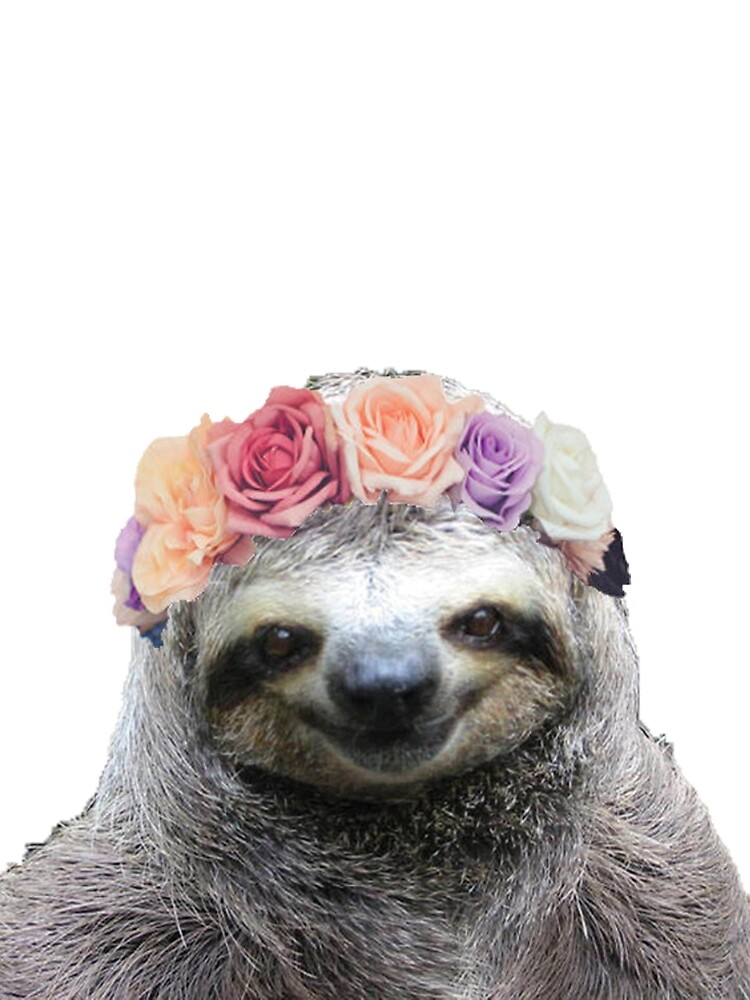The image is a detailed, square-format color photograph featuring a baby sloth's head and neck against a white background. The sloth appears to be smiling, with dark inset eyes and a bulbous black nose. Its fur is predominantly grayish-white, with darker areas and distinct black stripes extending from its eyes, creating a mask-like appearance. The sloth wears a crown of flowers, including purple, peach, pink, and white flowers, arranged across the top of its head in a seamless band without any greenery. The flowers blend naturally, suggesting a possible photoshop effect. The image captures the sloth from the top of its head to its mid-shoulders, emphasizing the contrast between the detailed, smiling sloth and the pure white backdrop. The photograph’s style is one of photographic representationalism and realism.